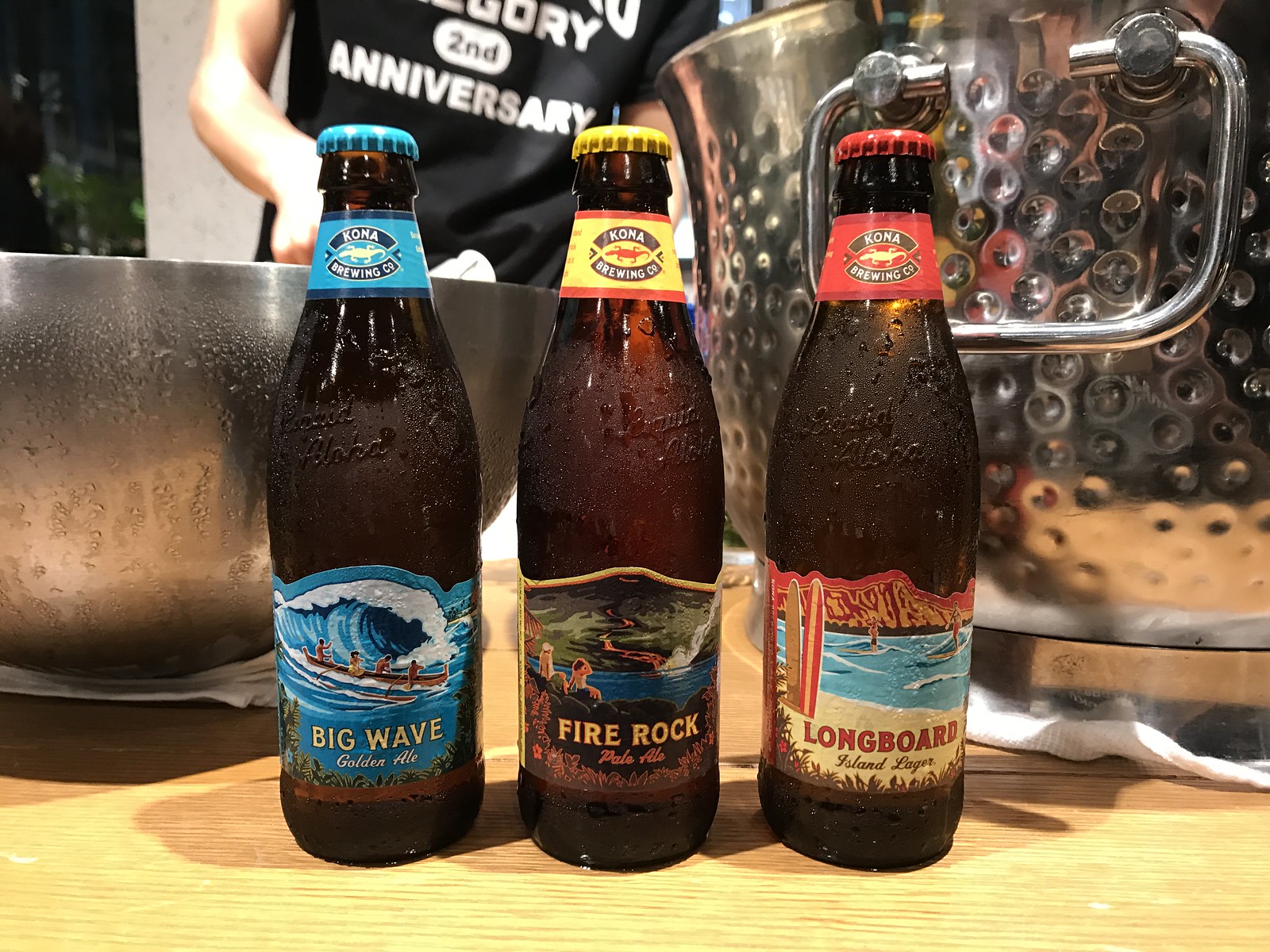In this detailed image, set in what appears to be the kitchen of a restaurant or bar, three ice-cold beer bottles are prominently displayed on a table. Each brown bottle is adorned with water droplets, hinting at their refreshing chill. In the background, blurred out of focus, a man in a black t-shirt with "Second Anniversary" in white lettering is seen cooking, surrounded by kitchen paraphernalia including large pots and a handled pan on a wooden countertop. To the left side of the image, a silver bucket, likely used for icing down drinks, adds to the scene's authentic feel.

The first beer bottle on the left, a dark brown bottle, has a blue cap and a vibrant blue label showcasing a Hawaiian scene. The label features a large Polynesian canoe paddled by four people against the backdrop of a towering wave, evoking the adventure of surfing. The label reads "Big Wave" in yellow, identifying it as Big Wave Golden Ale produced by Kona Brewing Co., with a distinctive lizard sticker on the neck.

The middle bottle, also dark brown, sports a yellow cap and a corresponding yellow label with the same Kona Brewing Co. branding. The label depicts an exciting volcanic scene where a stream of lava flows into the ocean, observed by two people. The text on the label reads "Fire Rock" in yellow at the top and "Pale Ale" in red below, enhancing the bottle's fiery theme.

The third bottle on the right has a red cap and matching red label. This label portrays a serene beach scene with mountains in the background and people paddleboarding across the surf. The text reads "Longboard Island Lager," suggesting a smooth, laid-back flavor. Like the others, this bottle carries the Kona Brewing Co. trademark lizard on the neck, cementing the surf-themed trio.

The cohesive imagery of surfing and Hawaiian landscapes across all three beer labels conveys a tropical, adventurous brand identity, appealing to those who love both craft beer and seaside adventures.